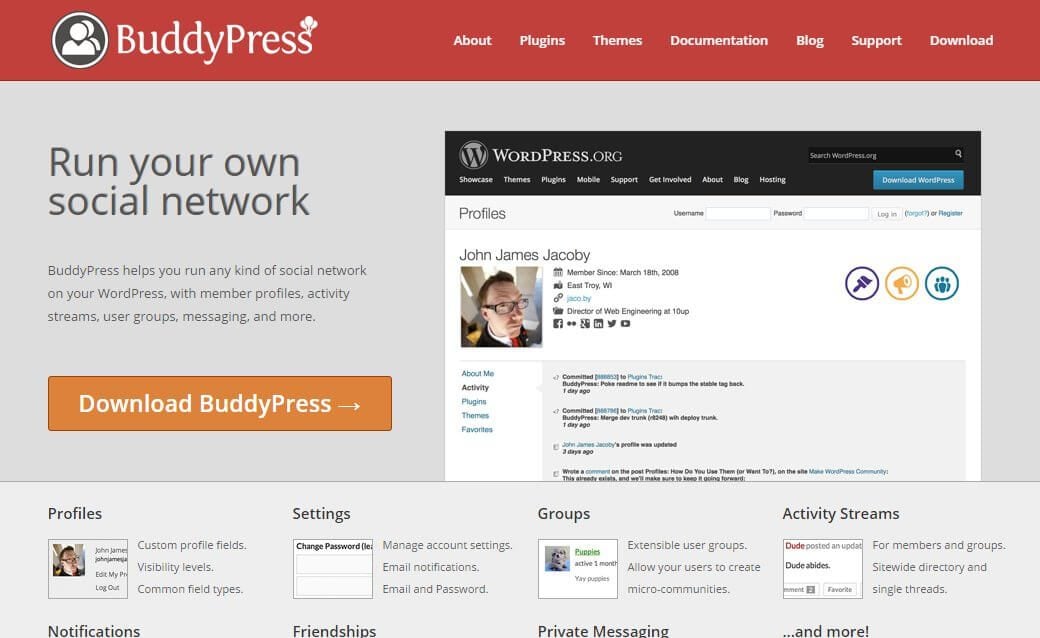The webpage being described belongs to BuddyPress, a WordPress plugin. At the very top of the page, there is a prominent red bar stretching across the screen. The logo is located on the left side of this bar, featuring a white icon depicting two human figures (one in front of the other) inside a gray circle with a white border, followed by the text "BuddyPress." On the final 's' of "BuddyPress," three small balloons are attached.

Below this, the top navigation bar provides several categories from left to right: About, Plugins, Themes, Documentation, Blog, Support, and Download. 

The main section of the page has a gray background. A prominent title toward the left side reads, "Run Your Own Social Network." Below this, in smaller text, is a tagline: "BuddyPress helps you run any kind of social network on your WordPress. There’s member profiles, activity streams, user groups, messaging, and more." Beneath these lines, there's an orange button labeled "Download BuddyPress" with an arrow pointing to the right.

To the right of this main content, there is an example mock-up of a WordPress profile page. At the top of this mock-up, a 'W' inside a circle is displayed, denoting the WordPress.org label with a search bar beneath it. The navigation options include Showcase, Themes, Plugins, Mobile, Support, Getting Involved, About, Blog, Hosting, and a blue "Download WordPress" button.

The profile section shows fields for Username, Password, and buttons for 'Login,' 'Forgot Password,' or 'Register.' There's an example profile for a user named John James Jacoby with details mentioning he has been a member since March 18, 2008, located in East Troy, Wisconsin. Additional profile information lists his role as the Director of Web Engineering at Ten Up.

Next to the profile details are multiple social media icons, suggesting connectivity to various platforms. Additional icons include a paintbrush in a white circle with a purple outline, a speakerphone in a white circle with a yellow outline, and three human icons within a blue outline.

Profile categories include About Me, Activity, Plugins, Themes, and Favorites. The 'Activity' section is selected, showing related content in a gray box.

At the very bottom of the page, several options are listed from left to right under different columns. The first column lists Profiles and Notifications, followed by Settings and Friendship. The next column lists Groups and Private Messaging, and the final column lists Activity Streams followed by "...and more!"

This detailed layout paints a comprehensive picture of both the BuddyPress service and its integration with WordPress.